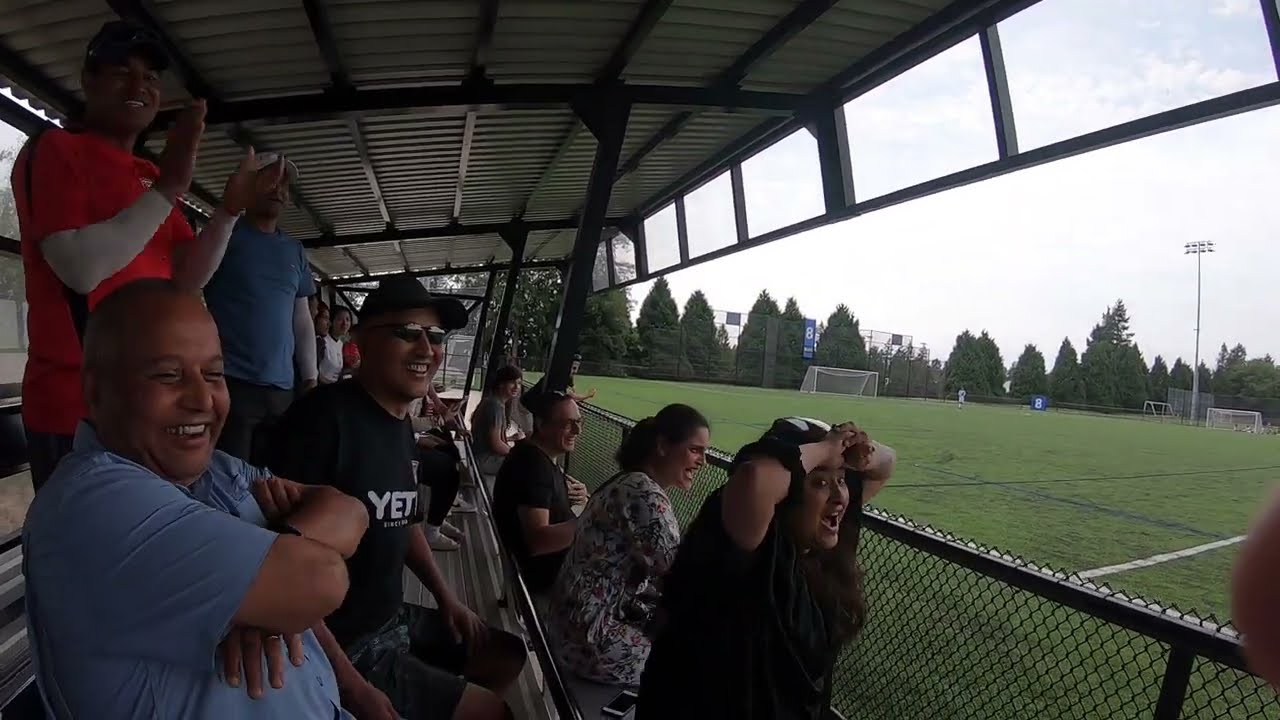The image captures a lively scene at a soccer match, where a group of 20 to 30 enthusiastic fans, both male and female, are seated in indoor stands under a metal awning. They are watching the action unfold on a large soccer field, which features white and blue lines marking various sections. A black chain link fence serves as a barrier between the spectators and the field. In the distance, the field is surrounded by rows of pine trees, creating a scenic backdrop, while multiple goalposts are visible, though only one player in white can be seen far off in the distance, possibly a goalie. There's also a blue banner displaying the number eight both up high and at ground level. The sky above is predominantly white, indicating it's a bright day, and a tall light pole stands in the area. The central focus is on the fans who are visibly enjoying the game, clapping, smiling, and capturing happy moments as they cheer for their team, suggesting a high-energy atmosphere. The fans' attire is diverse, ranging from blue to red, black, and white, enhancing the vibrant scene in this photograph.